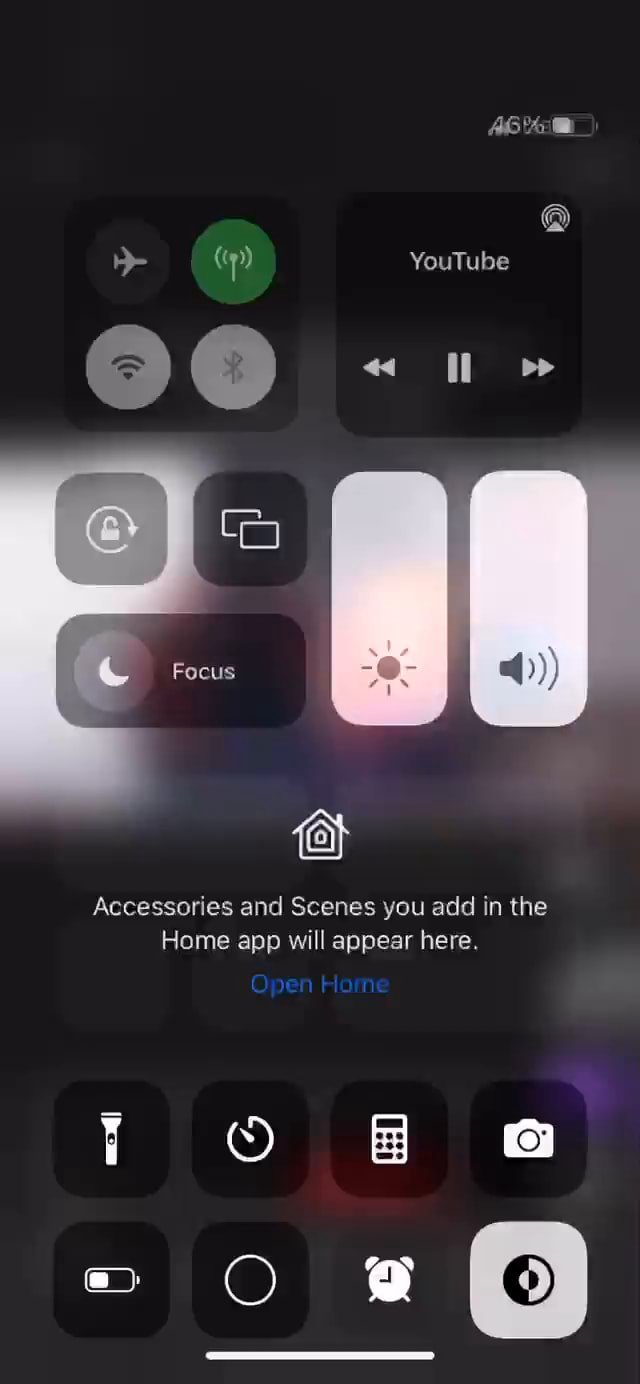This detailed caption describes a screenshot of a settings page from a mobile application with a styled layout focusing on functionality and accessibility.

---

The settings page is displayed against a blurred and darkened background, allowing the focus to remain on the content. The page is organized into a grid of tiles, each with a rectangular or square shape and rounded corners, making navigation intuitive.

- **Top-Left Tile**: 
  - A square, dark-colored tile divided into four sections, each containing a distinct icon:
    - **Top-Left Icon**: A white airplane on a dark-grey background, indicating airplane mode.
    - **Top-Right Icon**: A white telecom tower on a green background, possibly for network or signal settings.
    - **Bottom-Left Icon**: A medium-grey Wi-Fi symbol on a white background.
    - **Bottom-Right Icon**: A light-grey Bluetooth symbol within a white circle.

- **Top-Right Tile**: 
  - An identical background to the left tile, designated for media control. It features:
    - **Text**: "YouTube" centered at the top in white text.
    - **Media Controls**: Below the text are three buttons:
      - A white pause button in the center.
      - A white rewind button to the left.
      - A white fast-forward button to the right.

- **Middle-Right Section**:
  - Two vertical, white rectangles with rounded corners:
    - **Left Rectangle**: Contains a medium-grey sun icon at the bottom, suggesting brightness control.
    - **Right Rectangle**: Features a medium-grey speaker icon, indicating volume control.

- **Bottom Section**: To the left of the above tiles, structured as a combination of squares and a rectangle:
  - **Top Row**: Two side-by-side squares:
    - **Left Square**: A lock icon with a circular white arrow around it, possibly for screen rotation lock.
    - **Right Square**: Two stacked rectangular icons, suggesting some form of grouped settings or multi-window functionality.
  - **Bottom Rectangle**: Spanning the width of the two squares above, it displays:
    - **Left Side**: A medium-grey circle with a white crescent moon symbol, likely night or dark mode.
    - **Right Side**: The word "Focus" in white text, indicating a focus mode or do not disturb setting.

---

This structured and comprehensive caption encapsulates the visual attributes and inferred functionalities of the settings page, making it easy to visualize without the image.